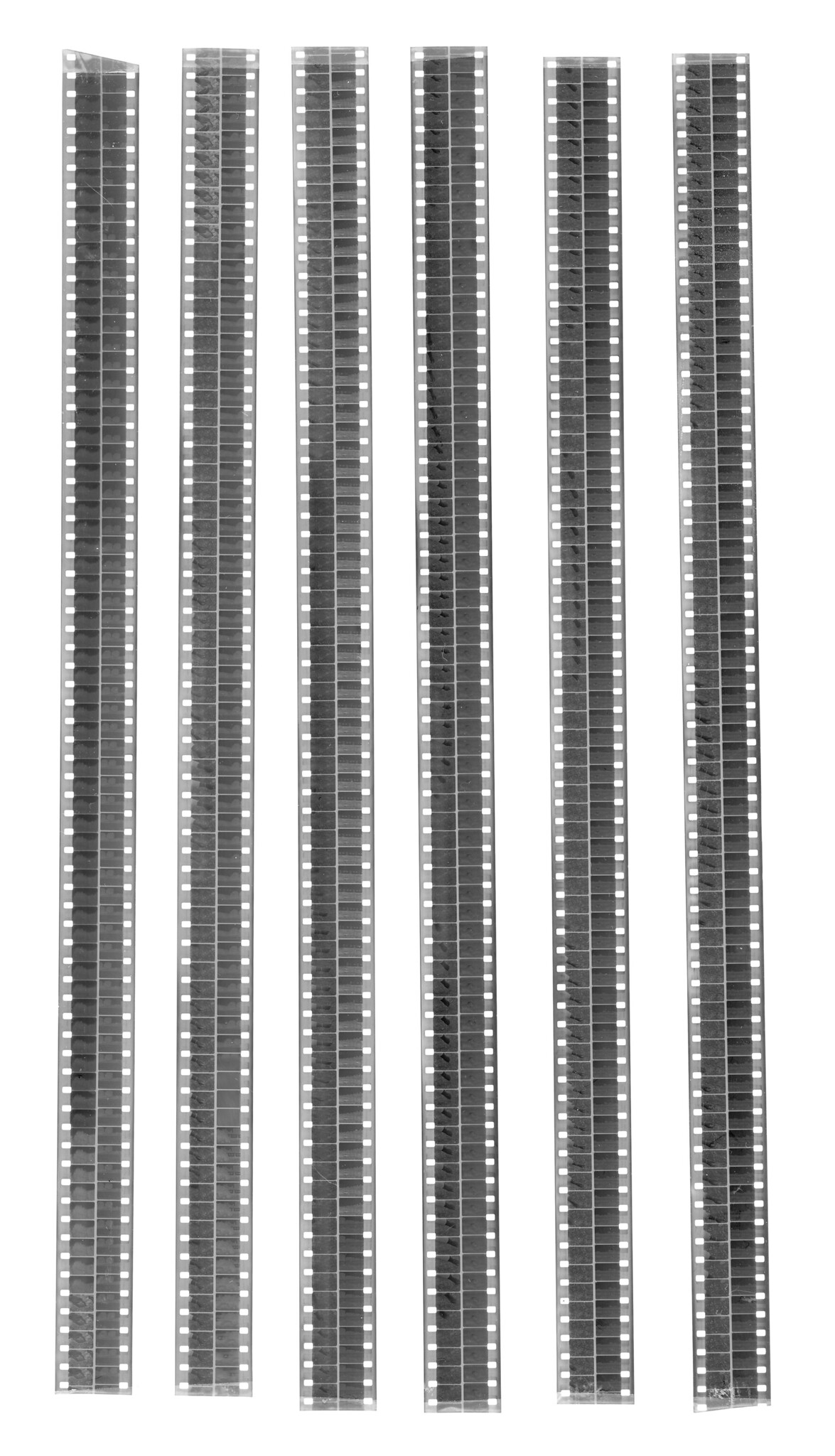This rectangular illustration features a basic black and white pattern devoid of any borders or photographs. The main design elements are six vertical strips that resemble film strips, each composed of little black squares with small white squares flanking either side. Between these film-like strips, solid white bands run vertically, creating a stark contrast. Each of the six strips varies slightly in shape and size: the first strip has a slanted top and a flat bottom; the second through fifth strips have both flat tops and bottoms but differ in height; and the sixth strip has a slanted bottom with a flat top. There are no pictures or text within the image, just a series of these meticulously arranged stripes, creating a repetitive yet nuanced pattern.